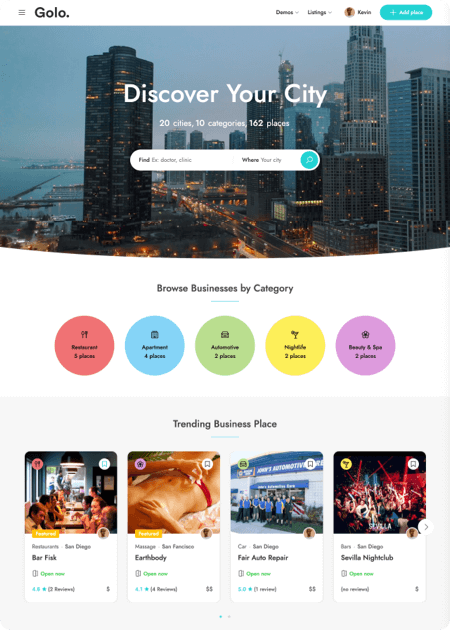**GOLO - Your Ultimate City Guide** 

The landing page for the GOLO website features a sleek design with user-friendly navigation tools. In the top left corner, the GOLO logo is prominently displayed alongside the three-bar menu icon, indicating expandable options.

The central focus of the page is a large, captivating image showcasing a city skyline with the text "Discover Your City" superimposed over it. This tagline emphasizes the site’s purpose as a city discovery and recommendation platform. Supporting this are the statistics displayed: "20 cities, 10 categories, 162 places."

Currently, user Kevin is signed in, with options such as "Listings" and "Add a Place" available. Below the main image, towards the middle of the page, users are prompted to search for specific businesses. Examples provided include doctor clinics, along with a "Where" and "What" input field paired with a magnifying glass icon for easy searching.

Just beneath this search section, a categorized browsing option is displayed:
- **Restaurants**: Represented by a pinkish-red circle with a fork and spoon icon, listing five places.
- **Apartments**: Marked by a light blue circle with an apartment building icon, showing four places.
- **Automotive**: Indicated by a light green circle with a car icon, featuring two places.
- **Nightlife**: Shown by a yellow circle with a martini glass icon, listing two places.
- **Beauty and Spa**: Represented by a light purple circle with a flower icon, listing two places.

Further down, the page highlights trending businesses in the current search area, which appears to be San Diego and San Francisco. Featured businesses include:
- **Bar Fisk**: A restaurant in San Diego, rated with four stars.
- **Earth Body**: A massage parlor in San Francisco, featuring a 4.1-star rating with numerous reviews. The image displays a woman's stomach, emphasizing relaxation services.
- **Fair Auto Repair**: Located in San Diego, this car repair service boasts a five-star rating, depicted with an image of people standing outside the shop.
- **Seville Nightclub**: A bar in San Diego without current reviews, shown with an image of patrons enjoying their time.

The page successfully provides a comprehensive guide to discovering city offerings across various categories, ensuring users can easily navigate and find relevant places and services.